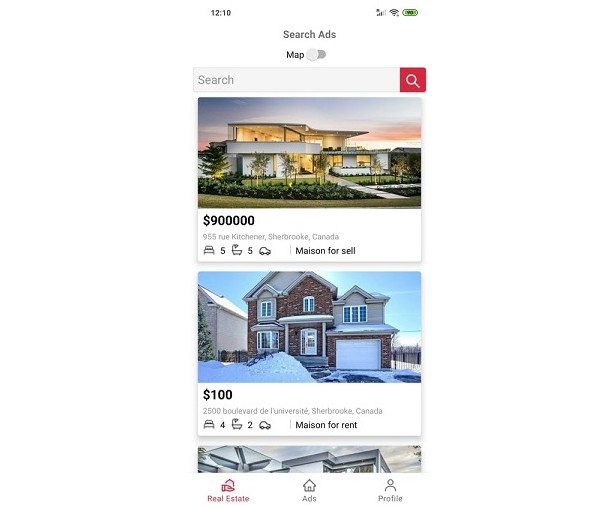The screenshot is taken from a cell phone and shows a real estate search interface at 12:10 PM. The phone battery is at 90%, and there are three bars of signal. The search heading reads "Search Ads" with the map feature turned off, focusing on the search box window displaying real estate listings. The top two listings are fully visible, while the third is partially cut off.

The first listing is for a house priced at $900,000, located at 955 Rue, Kitchener, Sherbrooke, Canada. The image shows a modern home with a flat roof, a balcony, and a neatly landscaped small front yard featuring a row of trees in front of a hedge, a shrubbery garden, plants, and a sidewalk.

The second listing is for a traditional two-story house, photographed in winter with snow piled around it. This house features a one and a half car garage, a beautiful front entryway with an early American look, a brick facade combined with wood siding, multi-pane windows, and a high peak above the second story. The listing price is erroneously displayed as $100, which doesn't match the home's described grandeur. This property is located at 2500 Boulevard D, University, Sherbrooke, Canada.

At the bottom of the screen, there are various navigation buttons labeled "MAISON," "real estate," "ads," and "profile," providing additional options for the user.